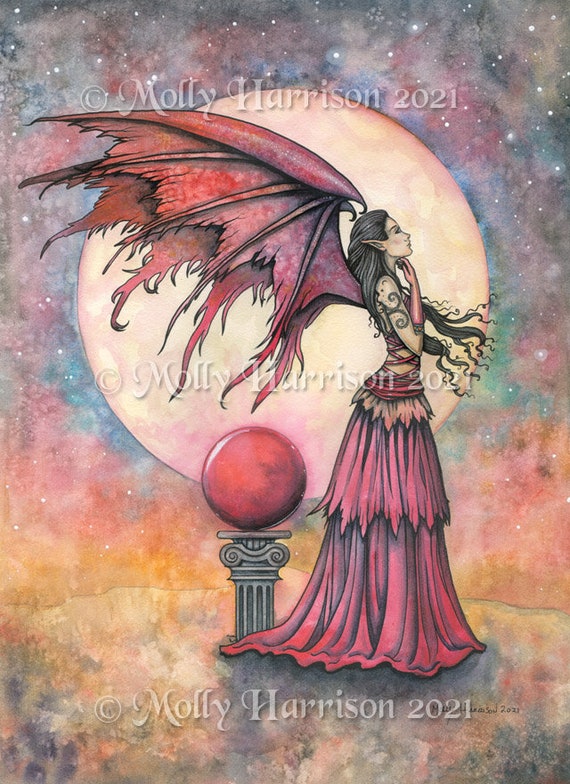This captivating vertical painting by Molly Harrison, titled "Copyright Molly Harrison 2021," presents an ethereal scene dominated by a fairy-like woman. The composition prominently features a large, glowing full moon in soft pastel hues of tan and pink, casting a gentle light on the scene. The woman, who gazes wistfully towards the upper right, is adorned with a flowing, two-tiered dress in muted shades of red and pink, its jagged edges adding a hint of wildness to her ethereal beauty. Her back is graced with extravagant red wings, textured with hints of black and gray that seem both delicate and powerful.

Her long, flowing black hair billows around her, with strands framing her delicate profile that showcases tall, pointed elf-like ears. Her right arm, visible and adorned with intricate black swirl tattoos, is bent slightly with her hand near her chin, adding to her contemplative demeanor. On her wrist, a matching red glove can be seen. 

Adding to the mystical ambiance, the background is a mesmerizing blend of reddish-purple and blue hues, speckled with star-like white spots that evoke a cosmic wonder. Behind her stands a marble pedestal topped with a radiant red orb, contributing to the image's dreamlike quality. The entire artwork bears the watermark "Molly Harrison 2021" thrice, in sheer whitish-gray lettering that subtly melds into the celestial background. This painting masterfully merges elements of fantasy and surreal beauty, leaving viewers enchanted by its detailed and mystical allure.